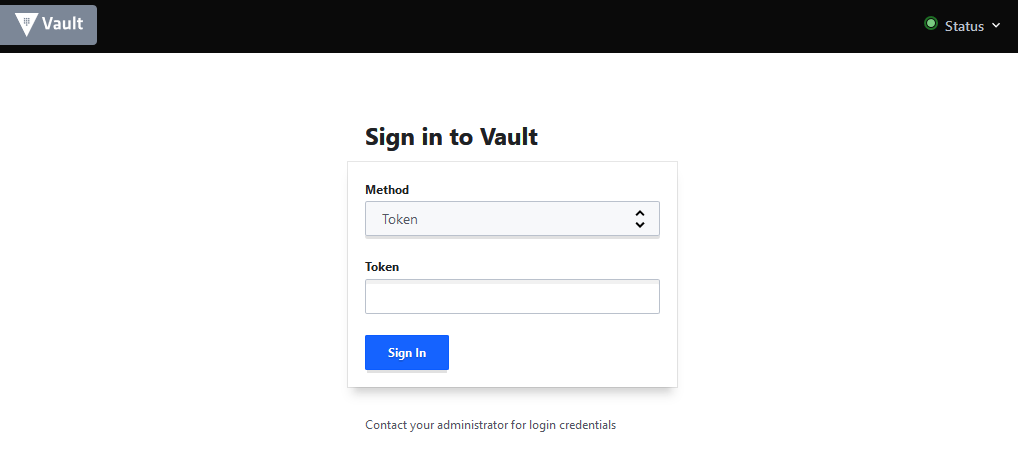The image is a screen capture of an application window with a white background. At the top, there is a black status bar. On the left side of the status bar, against a gray background, the word "Vault" is written in white, accompanied by an upside down white triangle to its left. On the right side of the status bar, also in white, is the word "Status" with a small green dot to its left.

Dominating the middle of the screen, in black text, are the words "Sign In to Vault." Below this, there is a dropdown button. On the upper left side of the dropdown button, the word "Method" is written in black. The dropdown button is currently displaying the word "Token" as the selected option.